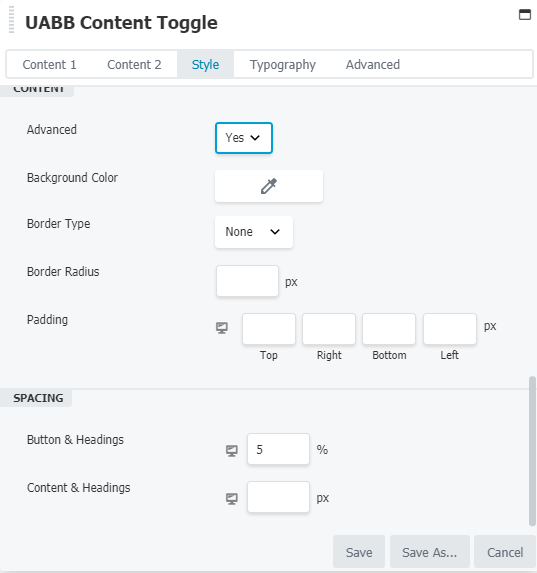The screenshot displays a portion of a webpage, specifically a utility page intended for configuring website settings. At the upper left corner, a black bold font reads "UABB" in all capital letters, followed by the words "content toggle." Below this header, there's a horizontal menu bar featuring several options: "Content 1" in gray font, "Content 2," and then "Style" highlighted in blue font against a light gray box, indicating it as the current selection. Following "Style," the options "Typography" in gray font on a white background, and "Advanced" are visible.

The background below the menu is a very pale blue, with a list of configuration options in gray font on the left side of the section. Each item is accompanied by a drop-down menu on its right. The items listed from top to bottom include "Advanced," "Background Color," "Border Type," "Border Radius," and "Padding." Below these configurations is another section labeled "Spacing," followed by "Buttons and Headings" and "Content and Headings."

In the lower right corner of the image, there are three buttons lined up horizontally: "Save" on the left, "Save As" in the middle, and "Cancel" on the right. This detailed layout indicates a settings configuration interface, designed for adjusting and saving various aspects of a website's appearance and behavior.